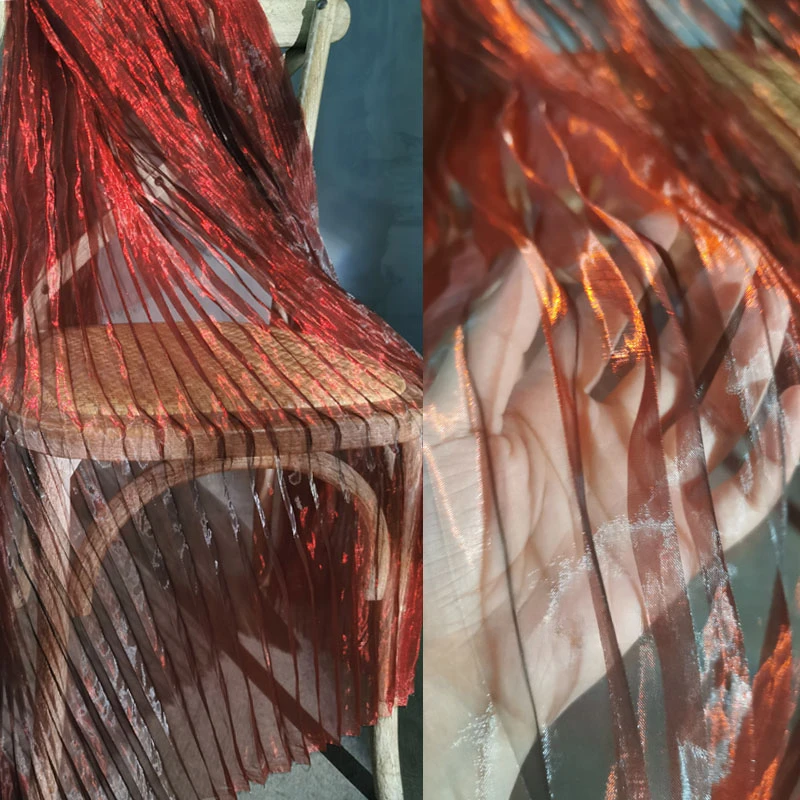The image consists of two side-by-side photographs, both featuring a piece of semi-transparent cloth with a reddish-orange tint. On the right side, a white person's hand, emerging from the bottom left, is partially visible just above the wrist, with the thumb and fingers naturally spread out, supporting the draped material that cascades over the fingers. On the left side, the same piece of fabric is elegantly draped over a wooden chair with a light green hue and a wicker cushion. The fabric covers most of the chair, descending from the upper left, leaving only the top right corner of the chair exposed. The setting appears to be in a neutral or grayish room.